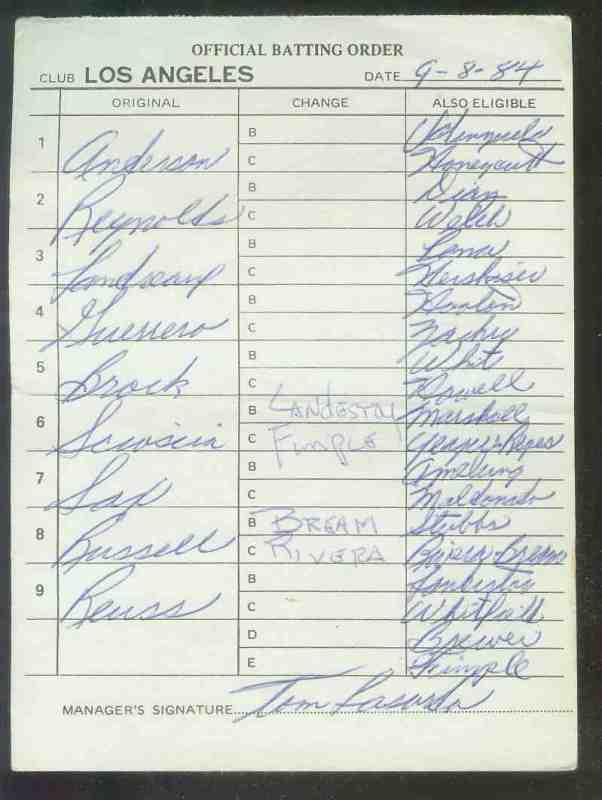This image features a sheet of paper that serves as an official batting order form for a baseball game. At the top, it prominently states "Official Batting Order" with "Club: Los Angeles" written on the left and the date "9-8-84" handwritten in blue ink on the right. The form appears to be old, with noticeable yellowing and creases indicative of age.

The main section is structured into a table featuring columns labeled "1 through 9" down the rows, "Original," "Change" (with sub-sections B and C), and "Also Eligible." Many of the cells in the "Change" column are blank, except for some printed letters in the sixth and eighth rows. The "Original" column contains a list of names written in the same loose, difficult-to-read cursive handwriting. Possible names include Anderson, Reynolds, Brock, Sanders, and Russell. In the "Also Eligible" column, names are inscribed in cursive as well.

At the bottom of the sheet, there is a section designated for the manager’s signature, which includes an inscrible text, potentially "Tim Frosch," written in blue ink. This signature is likewise in the loose cursive style seen throughout the document.